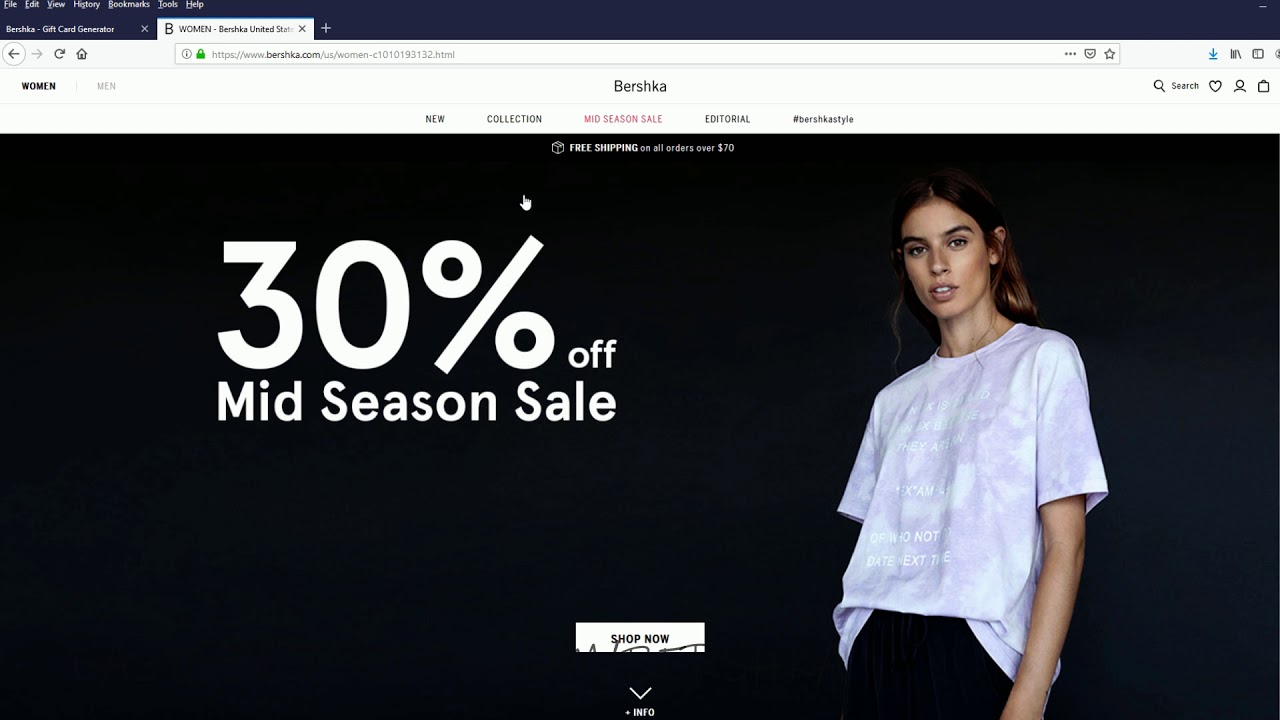The website for "Verishka" features a sleek and minimalistic landing page, primarily themed in black with stark white text. At the top of the page, there is a banner offering "Free Shipping on All Orders Over $70," highlighting a convenient shopping incentive. The focus of the page is the "Mid-Season Sale," prominently advertised with a large "30% Off" displayed in bold, eye-catching typography. Below this, the words "mid-season sale" are written in a slightly smaller font, both elements creating a dramatic contrast against the dark background.

Dominating the center of the page is a "Shop Now" button, enticing visitors to explore the discounts. Just above this call to action is a cursor pointer, drawing attention to interactive site elements.

A fashionably dressed model captures the viewer's gaze. The woman, who exudes an Eastern European aesthetic, is slender with brunette hair. She is dressed in a white patterned t-shirt, casually tucked in at the front, paired with black pants. Her pose, with hands in pockets and a nonchalant expression, adds to the chic and effortless vibe of the website, aligning with the overall brand image of "Verishka."